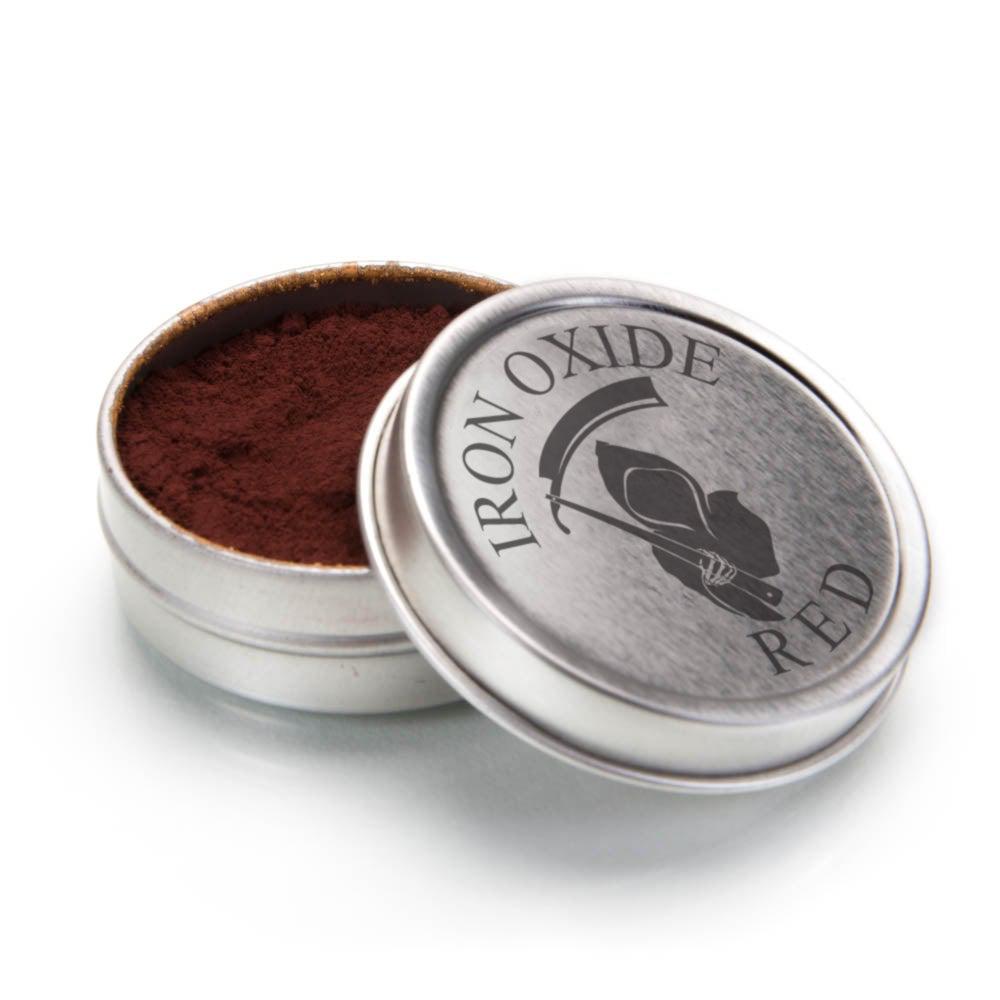The image depicts a silver tin can against a white background, with its lid leaning against it. The lid, marked with black text, reads "iron oxide red" and features a mysterious hooded figure holding a sickle above their head, resembling the Grim Reaper. Inside the tin, there's a noticeable reddish-brown powder, identified as iron oxide. Some of this powder is visible on the rim, and the rest fills the container, standing out vividly against the tin's metallic sheen.